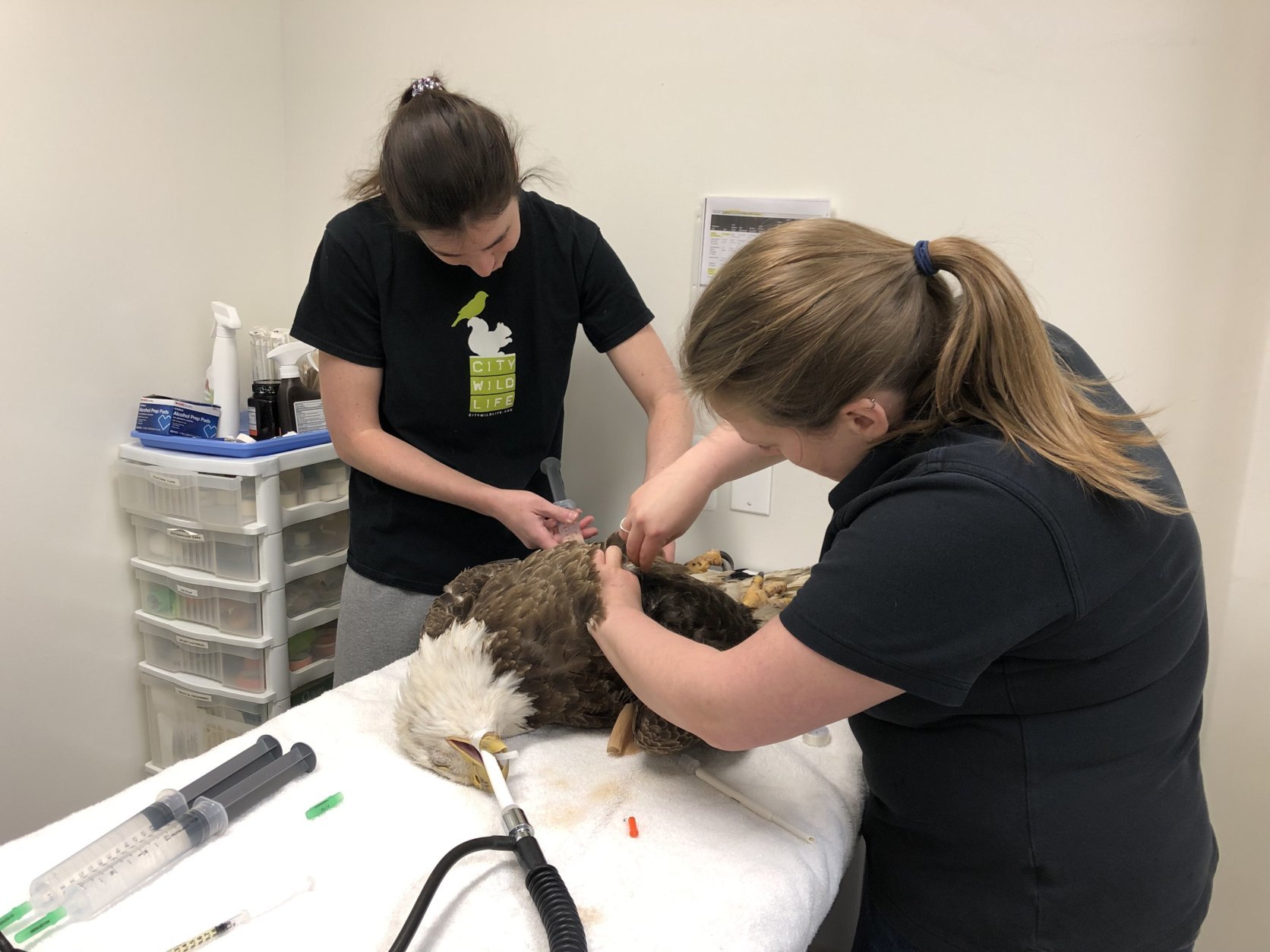In a pristine, white-walled veterinary room, two Caucasian female veterinarians are diligently working on a bald eagle laid out on a white operating table. The table is strewn with various medical instruments, including syringes. The eagle, sedated with a tube inserted into its mouth, appears to be undergoing an intricate medical procedure. The woman to the left, with dark brown hair tied in a ponytail and dressed in a black shirt and gray sweatpants, is holding a large syringe, with her left hand gently placed on the eagle's back. On the right stands a woman with sandy blonde hair, also in a ponytail and wearing a black shirt, her hands partly submerged in the eagle’s feathers as she attends to the bird's body. Behind them, a stack of clear plastic drawers containing medical supplies like gloves and spray bottles is visible, adding to the clinical atmosphere of the scene.